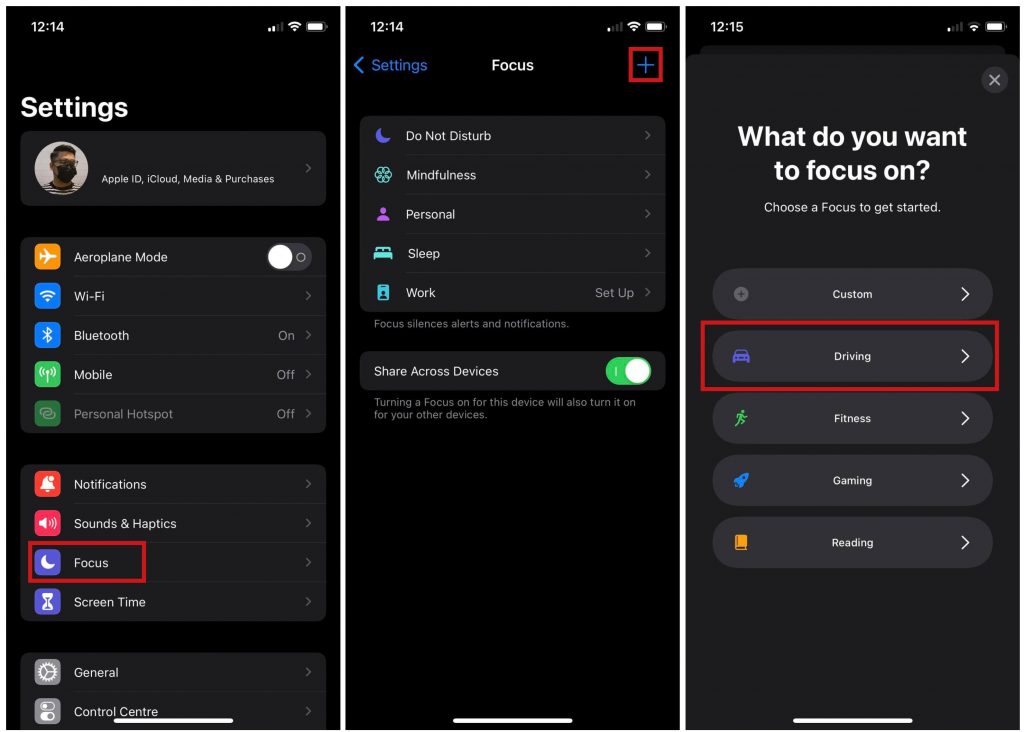The image depicts three individual smartphone screens, all displaying settings related to "Focus" modes. Here's a detailed breakdown of each screen:

**Left Screen:**
- **Top Bar:** Shows a time of 12:14. On the top right, there are icons for signal strength, Wi-Fi, and a nearly full battery.
- **Header:** The screen title "Settings" is displayed.
- **Profile Icon:** Positioned below the header.
- **First Section:** Lists options such as Airplane Mode, Wi-Fi, Bluetooth, Mobile Data, and Personal Hotspot.
- **Second Section:** Contains items like Notifications, Sound & Haptics, and Focus (highlighted with a red rectangle), followed by Screen Time.
- **Additional Options:** Below the second section are General and Control Center.

**Middle Screen:**
- **Top Bar:** Identical to the left screen, with a time of 12:14 and the same icons.
- **Header:** Displays "Settings" in blue, "Focus" in the center, and a blue plus sign on the right, highlighted with a red rectangle.
- **Focus Modes:** Lists various focus modes from top to bottom: Do Not Disturb, Mindfulness, Personal, Sleep, and Work.
- **Toggle Option:** Below the focus modes is an option labeled "Share Across Devices," which is enabled (indicated by a green and white button).

**Right Screen:**
- **Header:** Features a question in white text - "What do you want to focus on?"
- **Instruction:** Below the question, it says "Choose a Focus to get started."
- **Focus Options:** Lists five options for focus modes from top to bottom: Custom, Driving (highlighted with a red rectangle), Fitness, Gaming, and Reading.
- **Backgrounds:** All screens have a black background, while the individual options are displayed on grey backgrounds.

These screens collectively provide a detailed interface for managing various focus modes on a smartphone.